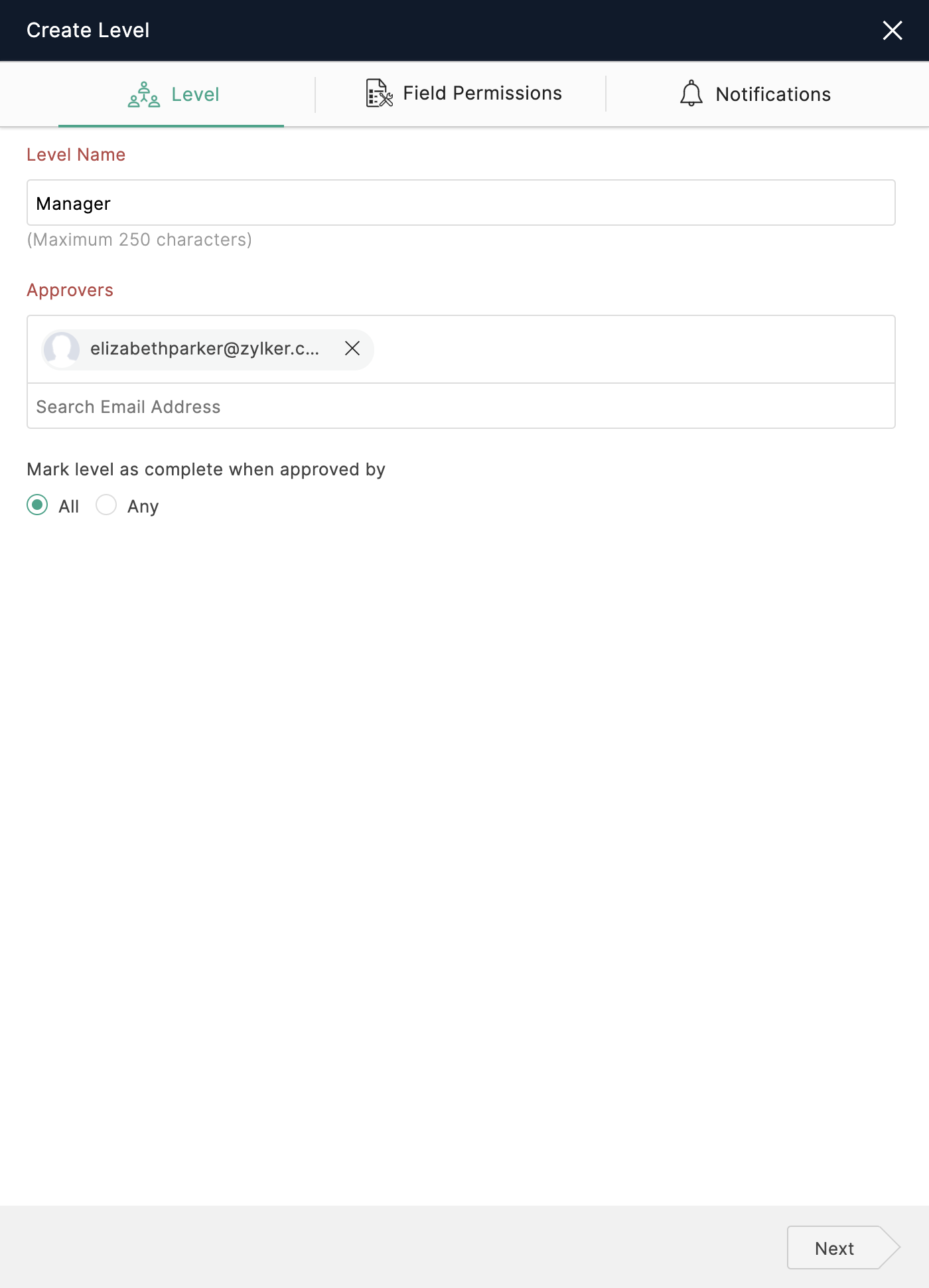In the image, we see a user interface for setting access levels and permissions within a platform. Key elements include fields for creating levels, setting field permissions, and configuring notifications. There is a text field labeled "Level Name" and an option to assign a manager. A note indicates that the maximum character limit is 250. Another field allows for entering approvers, exemplified by the placeholder "elizabethparkeratzilka.com," and a contextual hint to "search email address." There is a checkbox option "Mark level as complete when approved by all," followed by an option set to "Any."

At the bottom right corner of the interface, there is a "Next" button. Positioned at the top right corner is a "Close" button. The color scheme includes blue, white, black, and red, all set against a clean white background.